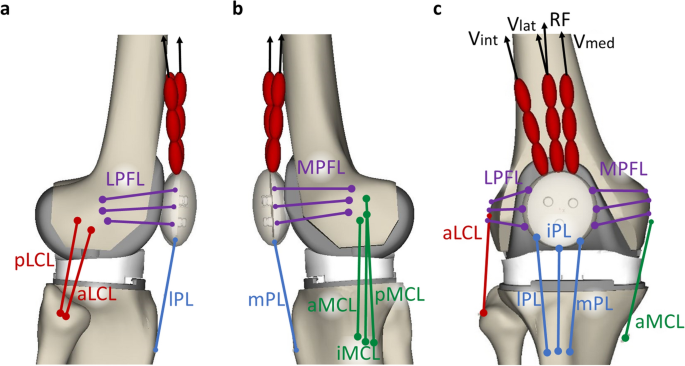The image is a detailed illustration of bone and joint structures, possibly representing knees or elbows. It contains three diagrams labeled A, B, and C, depicted from different perspectives: one from the right side, one from the left side, and one from the front. Each diagram illustrates bones in grey with black outlines and white connective tissues at the joint areas. The illustrations feature various colored labels and acronyms identifying different ligaments and anatomical features. The key labels include:

- From the front view, marked VINT and VLAT with red indicators pointing to what seem like small red round structures, possibly blood vessels or related structures.
- LPFL (Lateral Patellofemoral Ligament) and MPFL (Medial Patellofemoral Ligament) are labeled in purple at the knee area.
- RF (Rectus Femoris), V (Vastus), and VMED (Vastus Medialis) are indicated at the top with arrows.
- The side views label LPFL, MPFL, PLCL (Posterolateral Corner Ligament), ALCL (Anterolateral Corner Ligament), IPL (Inferior Patellar Ligament), MPL (Medial Patellar Ligament), and various MCLs (Medial Collateral Ligament) such as SMCL (Superficial MCL), AMCL (Anterior MCL), PMCL (Posterior MCL), and IMCL (Inferior MCL) in colors including purple, green, blue, and red.
- The bottom section labels include two bones at the leg's lower part, implied to be the tibia and fibula.

Overall, the diagrams are rich with annotations demonstrating an intricate mapping of the joint's ligaments and connective tissues, utilizing a color-coded system to differentiate each anatomical part.